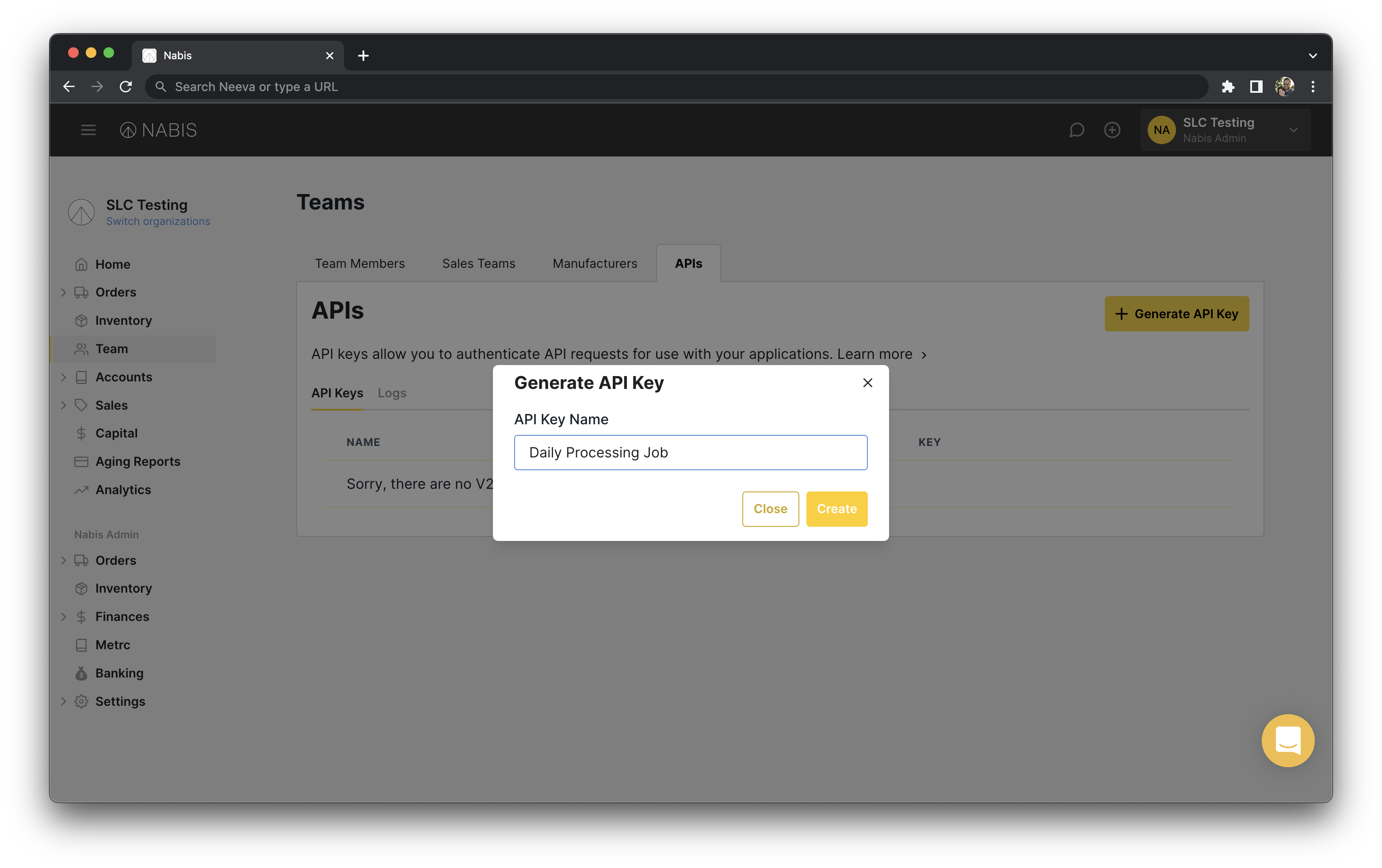A screenshot depicts a monochromatic black and gray website interface within a Microsoft Teams environment, focused on the generation of an API key for a daily processing job. The central part of the screen features a prominent modal window, overlaying and slightly dimming the rest of the page to draw attention to the API key creation process. This modal includes yellow-highlighted buttons labeled "Close," "Create," or "Generate," adding a touch of color and emphasizing user actions. The overall design appears utilitarian, underscoring the primary task of obtaining an API key, a security credential used for authentication in application programming interfaces.